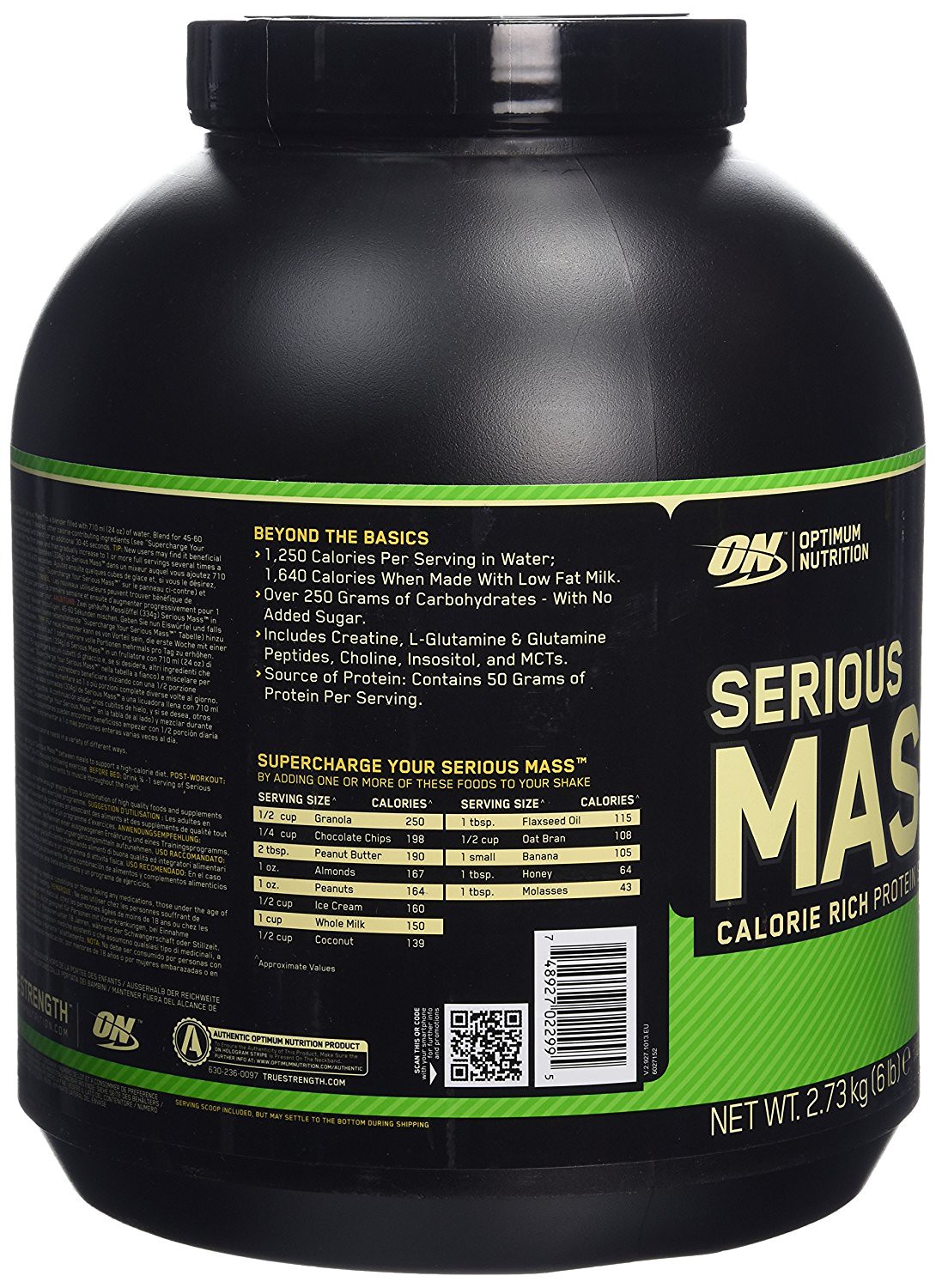The image features a compact, robust black bottle of a nutritional supplement. The bottle has a striking label in black and green, adorned with white lettering for clear visibility. Notably, on the back of the label, the phrase "Beyond the Basics" is prominently displayed. This supplement mix boasts a remarkable 1,250 calories per serving when mixed with water and is enriched with a rich protein content. Although the jar appears short and stout, it effectively conveys a sense of substantial volume with a net weight of 2.73 kilograms. Additionally, a barcode is visible on the back of the jar, accompanied by a QR code for seamless access to the manufacturer's website for further information.